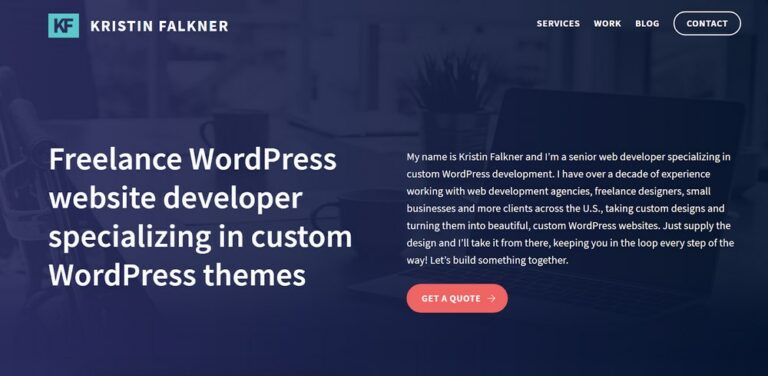Shown is a sophisticated digital advertisement for a freelance WordPress website developer. The ad features a dark blue background with a lighter blue design resembling a laptop, accompanied by two mugs, a plant, and faint window visuals in the background, creating a cozy yet professional ambiance.

In the top left corner, a teal rectangle houses the initials "KF" in dark blue letters. To the right of this logo, "Kristin Faulkner" is boldly displayed in all caps with the first and last names clearly spelled out.

The upper right section presents three navigational links—"SERVICES," "WORK," and "BLOG"—in white, all-caps, bold letters. Adjacent to these links is a rounded rectangular button with a dark blue interior and white border that reads "CONTACT" in white letters.

Centered within the ad, large white text proclaims, "FREELANCE WORDPRESS WEBSITE DEVELOPER SPECIALIZING IN CUSTOM WORDPRESS THEMES." Below, a detailed introduction reads, "My name is Kristin Faulkner, and I am a senior web developer specializing in custom WordPress development. I have over a decade of experience working with web development agencies, freelance designers, small businesses, and more clients across the U.S., taking custom designs and turning them into beautiful, custom WordPress websites. Just supply the design and I'll take it from there, keeping you in the loop every step of the way! Let's build something together."

At the bottom, a pinkish-red rectangular button with rounded corners stands out, featuring bold white text that says "GET A QUOTE" along with a right-pointing arrow, inviting viewers to take the next step.